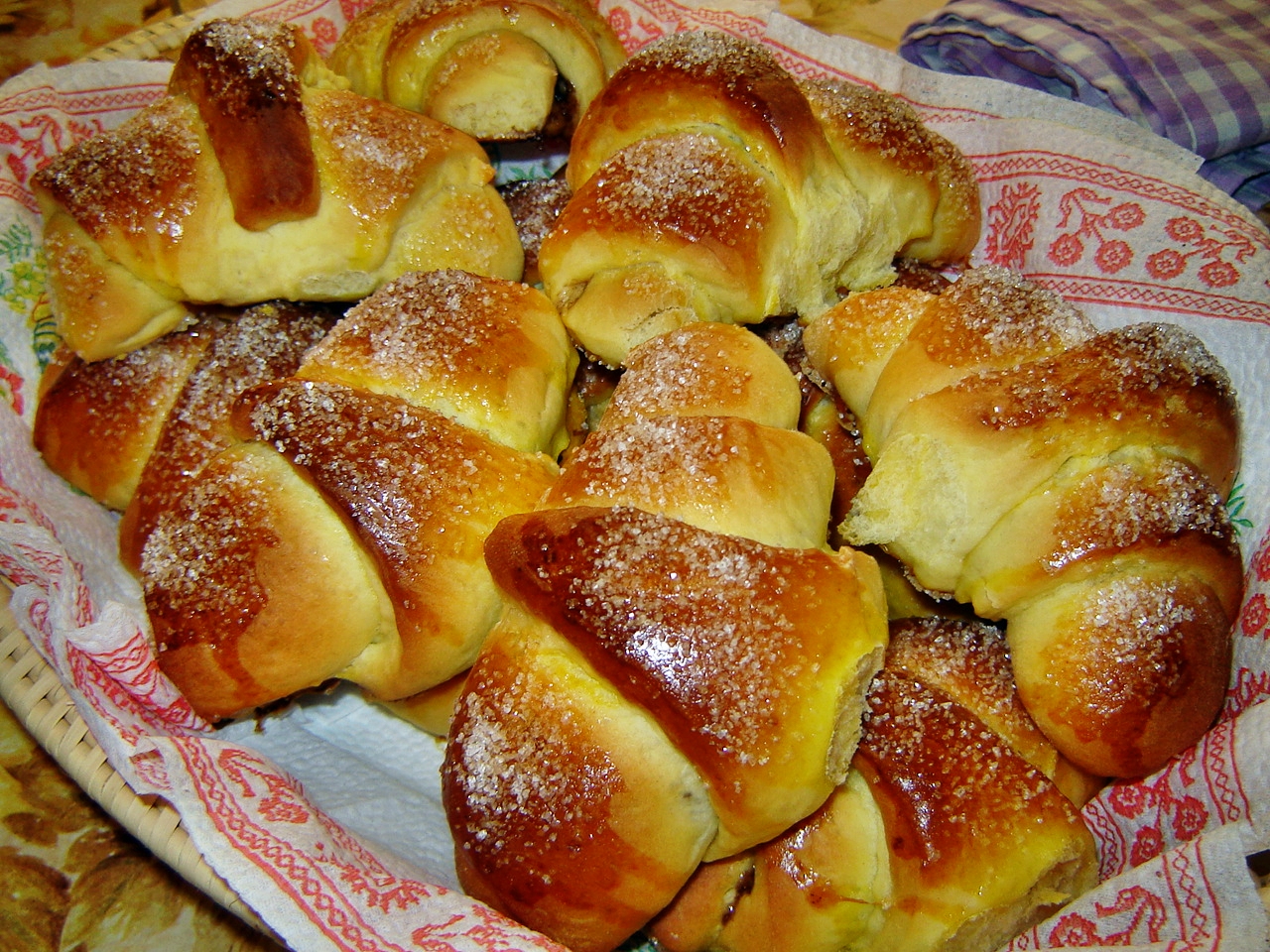This horizontal rectangular image showcases a bountiful plate of freshly baked rolls, nearly hidden under a white napkin with a distinctive orange border. The plate itself, glimpsed through the napkin, is edged in brown. The rolls, which resemble butter rolls shaped like croissants, are golden yellow with dark brown tops, glistening with a sprinkling of salt. They fill the plate abundantly, their shiny surfaces hinting at a buttery, perhaps slightly sugary coating. The setup suggests a serving style suitable for a cozy restaurant, enhancing the homely yet elegant presentation.